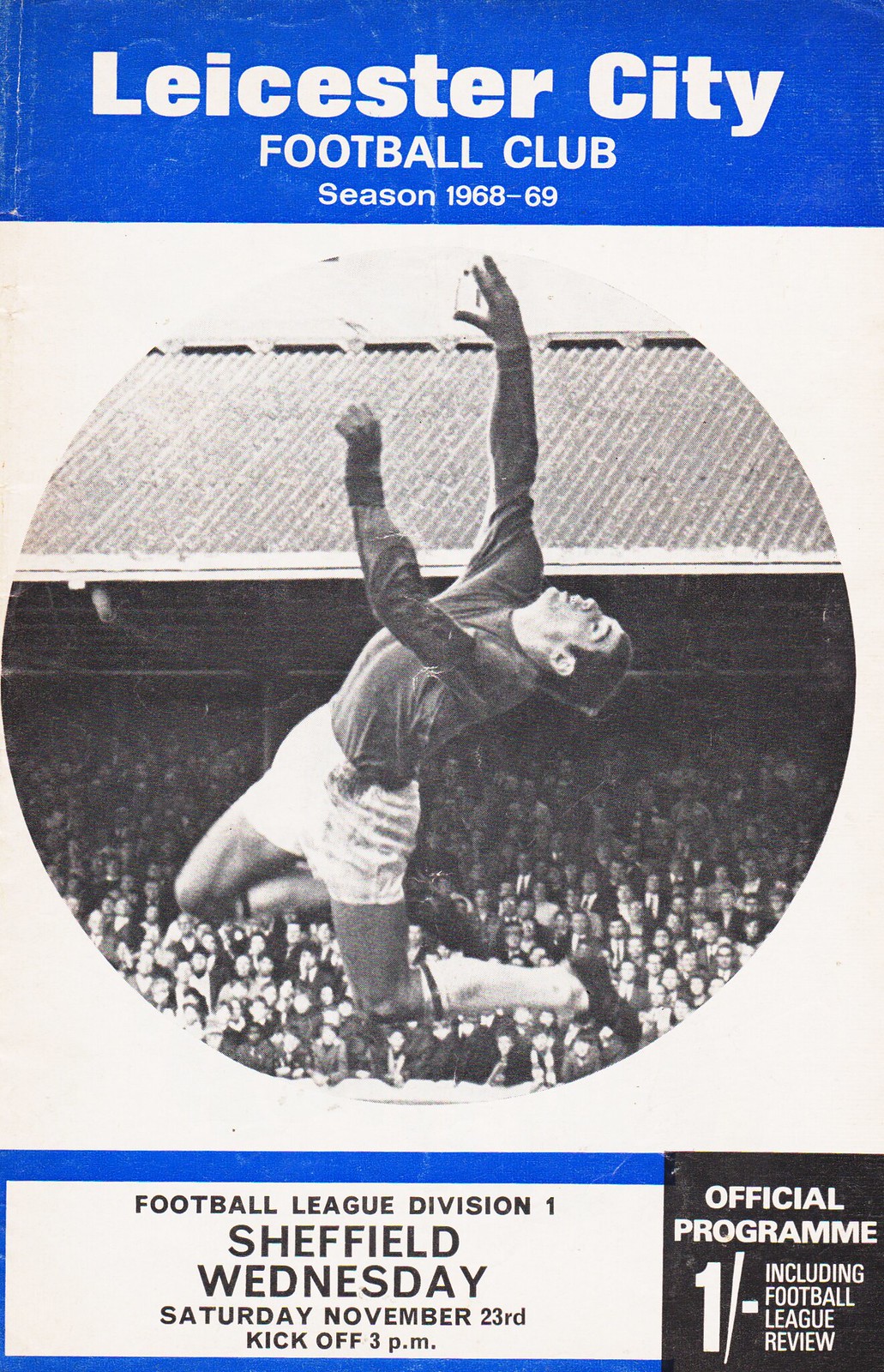The image is the front cover of an official program from the Leicester City Football Club for the 1968-69 season. Across the top, in bold blue text, it reads "Leicester City Football Club, Season 1968-69." Centrally placed is a round, black-and-white photo of a football player dressed in a long-sleeve sweatshirt, white shorts, knee-high socks, and black shoes, with a crowd in the background. Below the photo, the text announces "Football League, Division 1, Sheffield Wednesday, Saturday, November 23rd, kickoff, 3pm." In the lower right-hand corner, it states, "Official Program 1, including Football League Review." The cover features a classic design typical of vintage match-day programs, employing a color scheme of blue, white, off-white, black, and various shades of grey.